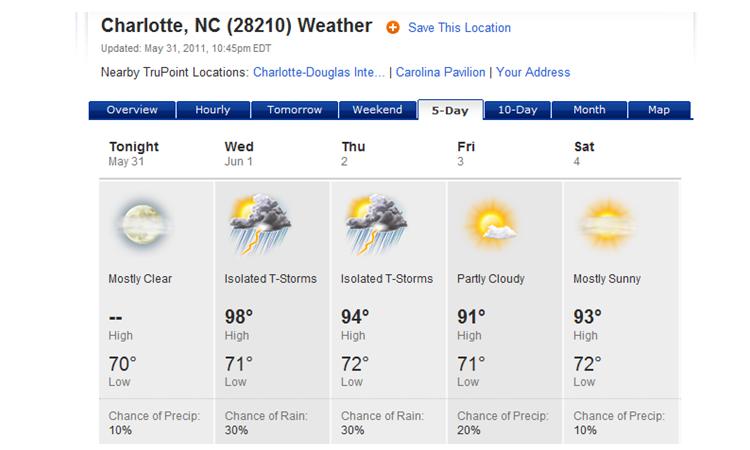**Detailed Weather Forecast for Charlotte, NC (28210)**

*Updated May 31, 2011, 10:45 PM*

Navigate to:
- Overview
- Hourly
- Tomorrow
- Weekend
- 5-Day
- 10-Day
- Month
- Map

**Current Weather:**
- **Tonight, May 31st:** Mostly clear skies with a low of 70°F. Slight chance of precipitation at 10%. (Icon: Moon with partial cloud cover)

**5-Day Weather Forecast:**
- **Wednesday, June 1st:** Expect isolated thunderstorms throughout the day. High of 98°F and a low of 71°F. (Icon: Sun behind storm clouds)
- **Thursday, June 2nd:** Continued isolated thunderstorms with a high of 95°F and a low of 72°F.
- **Friday, June 3rd:** Partly cloudy skies with a high of 91°F and a low of 71°F. (Icon: Sun with a small cloud)
- **Saturday, June 4th:** Mostly sunny conditions with a high of 93°F and a low of 72°F.

**Nearby True Point Locations:**
- Charlotte Douglas International
- Charlotte Carolina Pavilion
- Your Address

(Note: The 5-day forecast is highlighted in a white bar with black letters.)